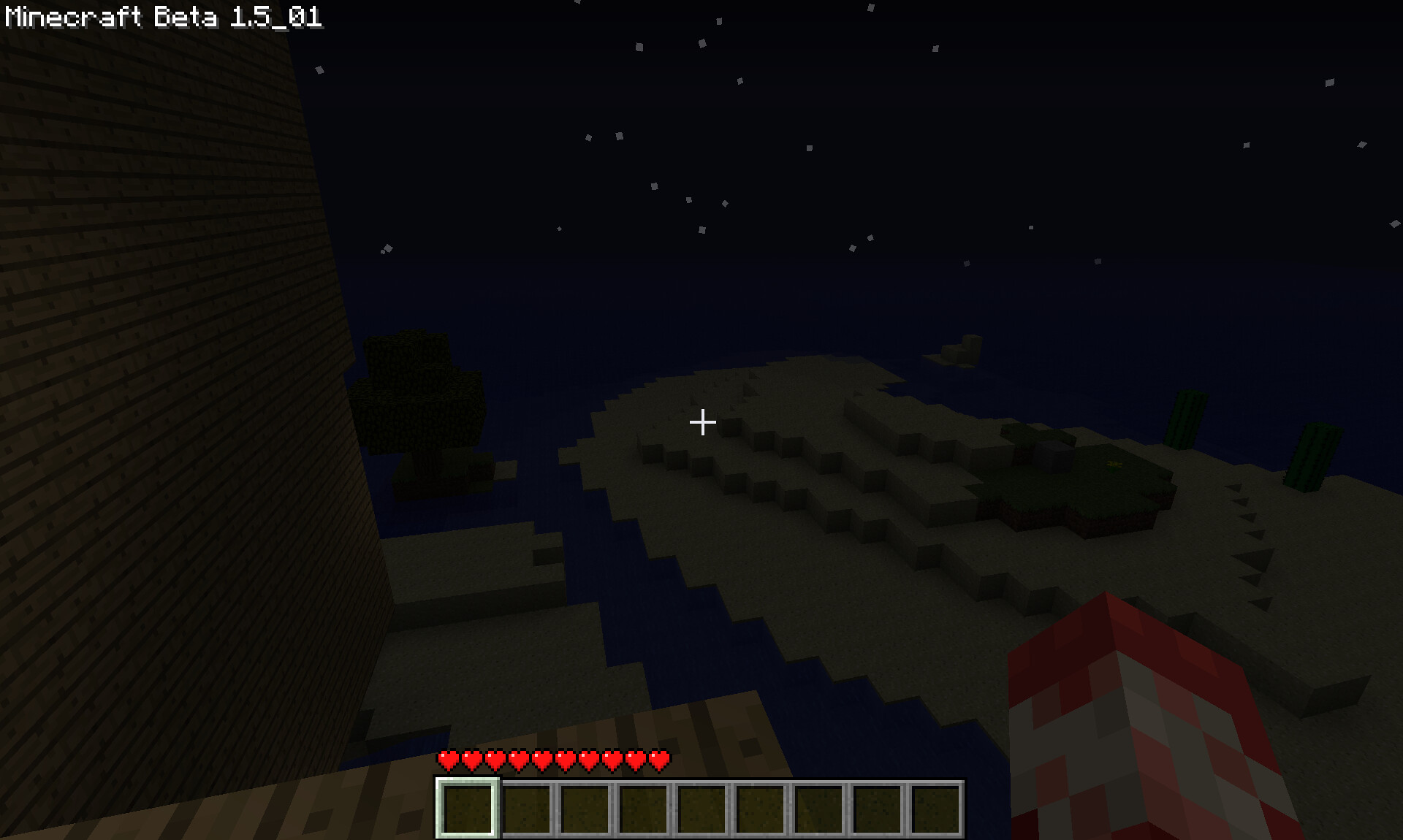This is a screenshot from Minecraft Beta 1.5_01 taken at night, featuring a dark black sky speckled with small, gray stars. Prominently displayed in white text at the upper-left corner of the screen is the version information: "Minecraft Beta 1.5_01". The bottom area of the image shows the Minecraft HUD, a series of nine gray, square sections indicating the inventory slots. Just above these slots, there is a row of red hearts denoting the player's hit points or health.

In the center of the picture, there's a white plus sign functioning as a crosshair. On the left-hand side, a structure made up of brick-like blocks is visible, while further towards the center, there’s an alternating pattern of red, gray, pink, and dark pink stones, suggesting another building section or wall.

To the right side of the image, a reddish block is noticeable, likely the player's hand, commonly seen in first-person perspective games. In the distance, elements of the game's landscape such as blocks resembling an ocean and surrounding hills can be vaguely seen, as well as tall trees on what appears to be an island, all composed of Minecraft’s signature low-resolution blocks.